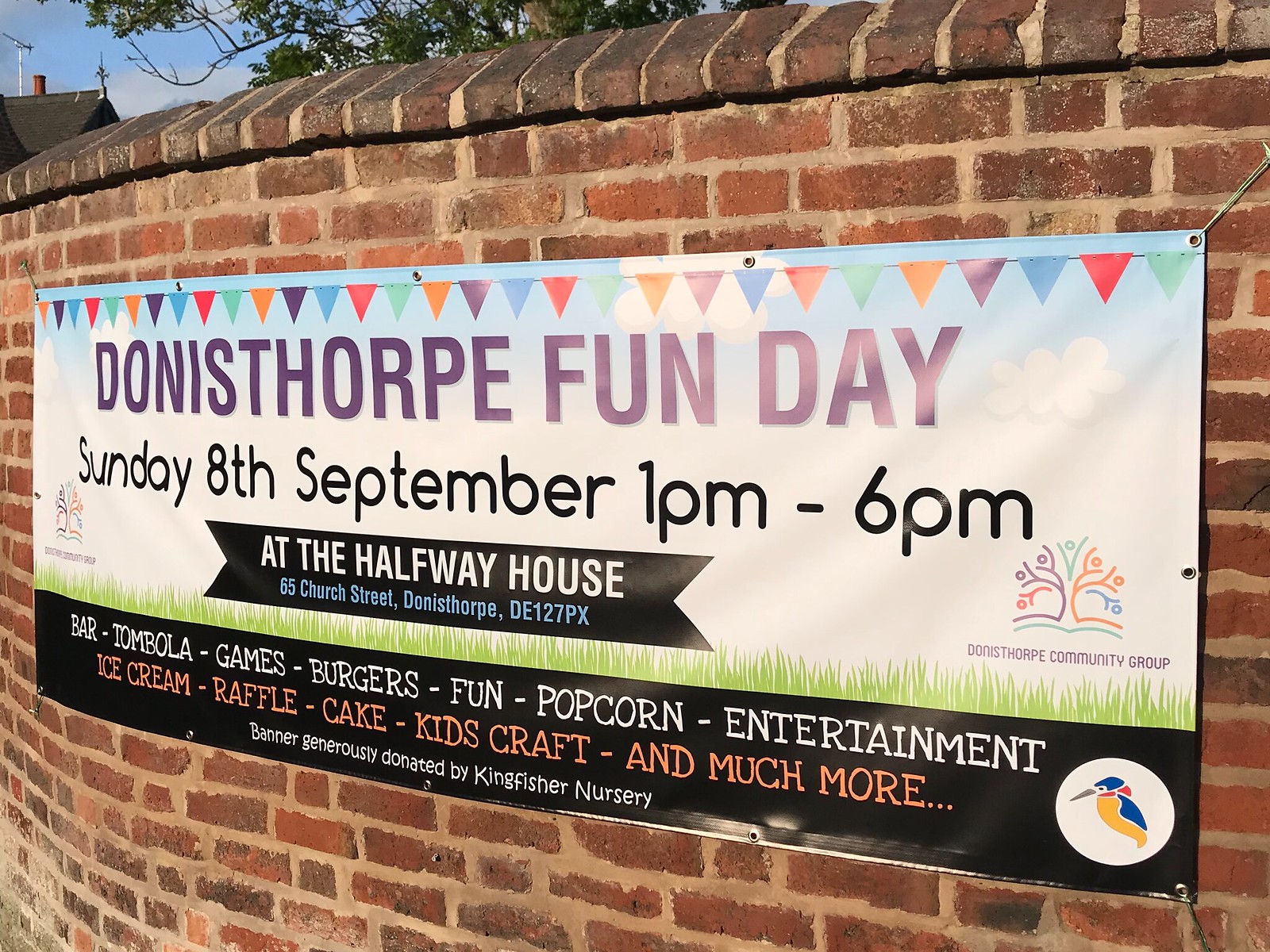The image showcases an aged, curved brick wall that serves as a barrier or fence, possibly part of an old guard wall. Mounted on this wall is a vividly designed tarpaulin banner featuring a blue sky with white clouds and a green grass backdrop, adorned with decorative ribbons and a colorful stream of triangular flags. The banner announces the "Donisthorpe Fun Day" in large purple text, followed by the event details in smaller black text: "Sunday 8th September, 1 p.m. to 6 p.m." Below, a black ribbon-styled box contains the text "at the Halfway House, 65 Church Street, Donisthorpe DE 127 PX," accompanied by a vibrant logo of a tree with children jumping in orange, green, and purple hues on both the left and right corners. The bottom section of the banner, bordered by a black bar, lists activities such as a bar, tombola, games, burgers, fun, popcorn, entertainment, ice cream, raffle, cake, kids crafts, and much more. The banner specifies that it was generously donated by Kingfisher Nursery, whose logo is depicted inside a white circle at the bottom right corner. The background includes the silhouette of a tree with branches and leaves peeking over the wall, a clear blue sky, and the roof and chimney of a nearby house visible in the top left corner of the image.